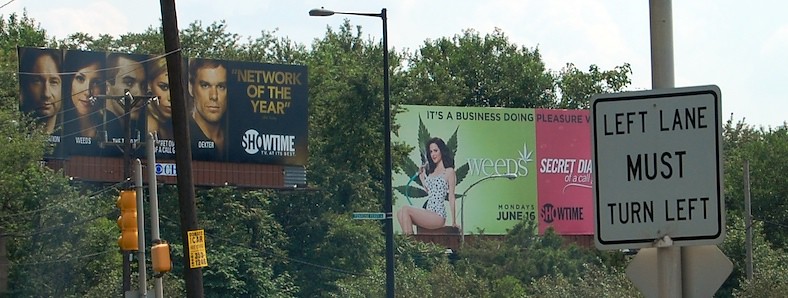Under a moody gray sky, an urban landscape unfolds. Interspersed with clusters of trees bearing thick green leaves, a noticeable black billboard stands prominently on the left side of the image. This billboard, belonging to CBS, features actor names at the bottom, with “Showtime” inscribed on the bottom right. The upper right corner bears the accolades "Network of the Year" and "Connelly Golden."

To the right of this, another billboard makes a striking statement with "It’s a Business Doing Pleasure" written across it. The left side of this sign features the word “Weeds,” whereas the right side mentions the "Secret Diaries of Paul [last name indistinct]." At the bottom, it announces a significant date: "Monday, June 16th," accompanied by the Showtime logo on the right.

Further right, a traffic directive informs drivers with a sign saying, "Left Lane Must Turn Left." Beside it, wooden poles punctuate the scene, further enhancing the image of this functional yet picturesque streetscape.